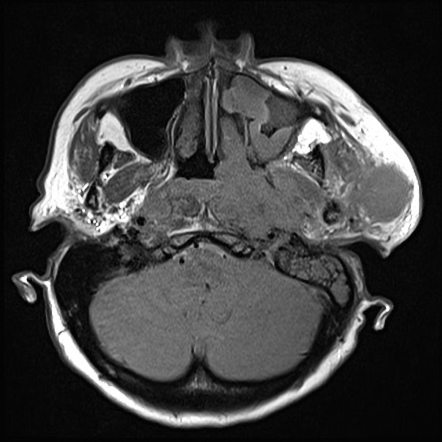The monochrome grayscale image displays a highly detailed, complex structure resembling an internal body part, possibly from an animal. Set against a solid black background, the lower part of the image showcases a white outline enclosing an upside-down heart-shaped object in shades of gray. The intricate composition of what appears to be muscles and organs can be seen at the top of the image, denoted in varying shades of gray. The outer edge of the structure is delineated in white, suggesting a skeletal boundary, and features three protruding bones at the top, which could be likened to shoulders. The design within the structure is symmetrically intricate, with black spaces on the left, a large blotch of white on the left, and smaller blotches of gray and white on the right side. The internal patterns, grooves, and dots in gray, black, and white give the appearance of something organic, like an embryo or a detailed x-ray of internal organs, or alternatively a piece of intricately shaped steel.